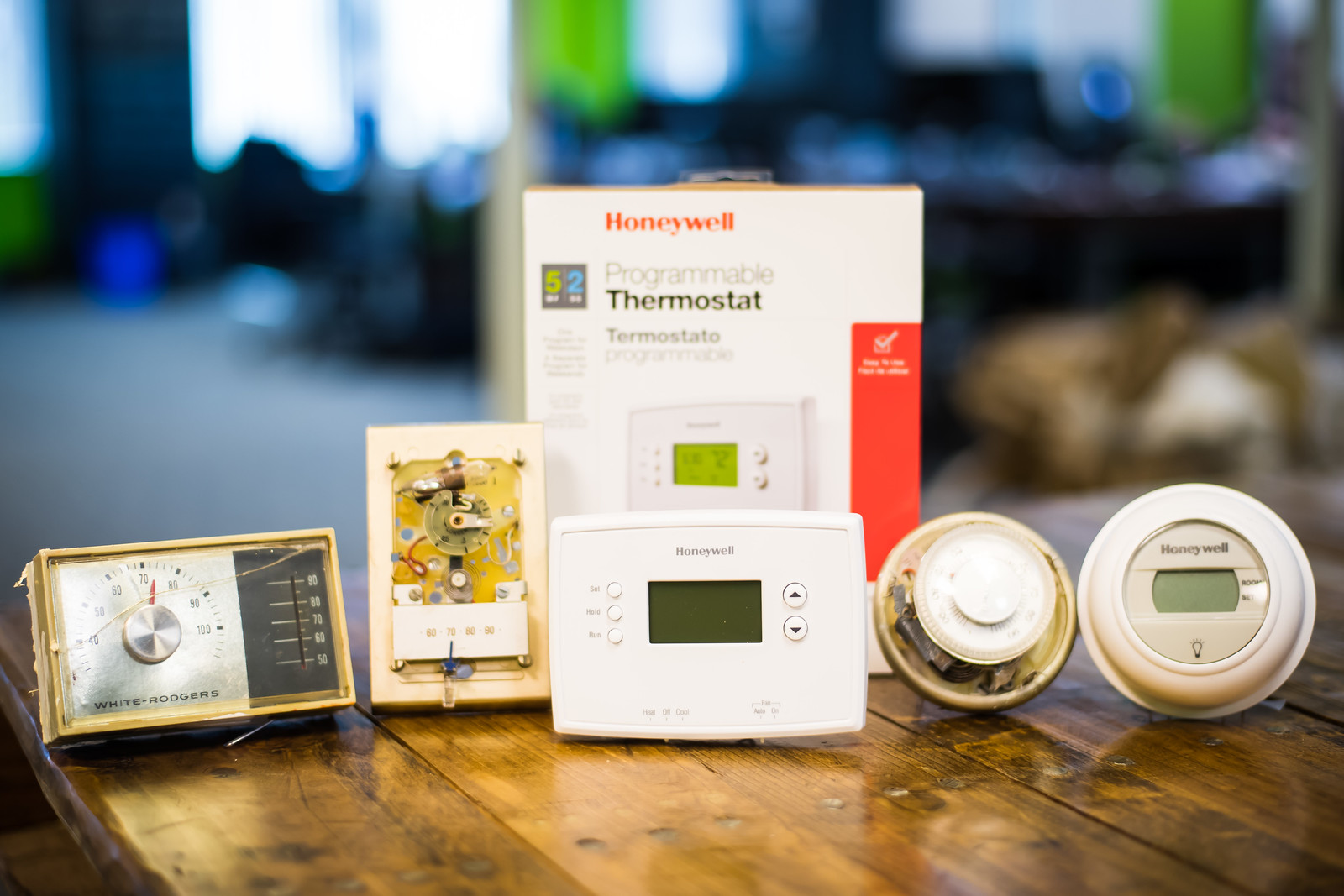This image showcases an array of five thermostats spanning different eras, aligned side by side on the surface of what resembles a wooden picnic table. The table's corner is visible in the lower left portion of the image, angled towards the center. On the far left, there is a square thermostat equipped with a turn knob. Adjacent to it is a classic mercury thermostat with a visible internal thermometer and a lever at the bottom for manual adjustment. The middle of the lineup features a modern Honeywell LED thermostat, still in its original packaging. To its right sits another turn-type thermostat; however, the central mechanism is missing, leaving only the front knob visible. Completing the row is a contemporary Honeywell LED digital thermostat, highlighting the evolution of thermostat technology in both design and functionality.